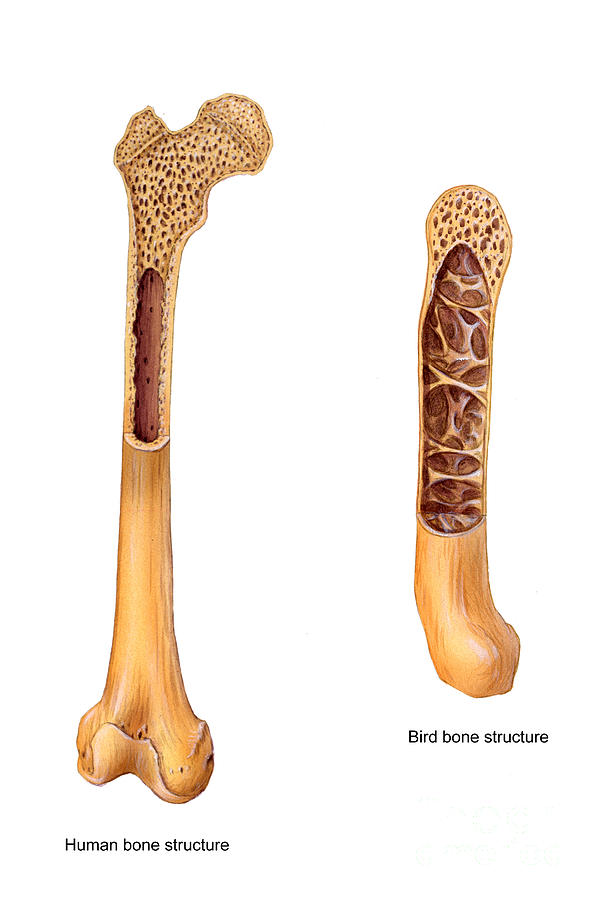The image is a detailed medical illustration comparing the bone structures of a human and a bird. Rendered primarily in tan and brown with touches of white, the illustration features two distinct bones. The human bone, which is long and slender, has a cutaway section at its top revealing its internal composition: spongy texture with a hollow middle. In contrast, the bird bone is shorter and thicker with a notably different architecture. Its internal structure is characterized by numerous air pockets and significantly less dense bone. This comparative anatomy illustration, likely from a textbook in zoology or a related field, highlights the anatomical differences and similarities between the two species, showcasing the human bone's elongated, narrower form versus the bird bone's more detailed, hollow design.